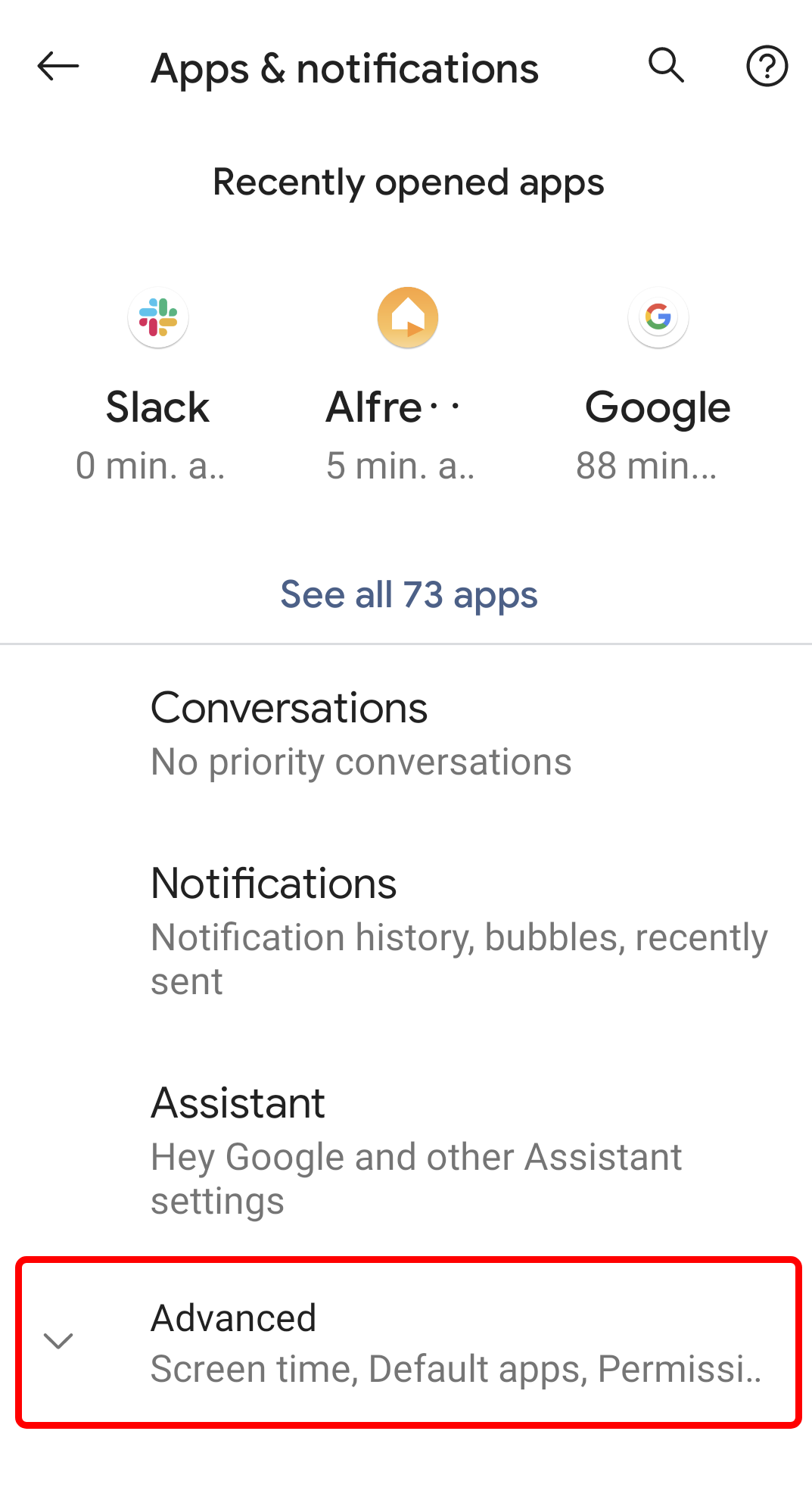A detailed screenshot of a mobile device settings page is displayed, specifically within the "Apps and Notifications" section. The interface is characterized by a clean white background, with a navigation arrow located at the top left corner. Adjacent to it, the header reads "Apps and Notifications," flanked by a magnifying glass icon and a help icon (a question mark inside a circle).

Directly beneath the header, the screen lists "Recently Opened Apps," including:
- Slack, with a usage time of 0 minutes.
- An app abbreviated as "I.A.L.F.R.E," used for 5 minutes, with ellipses following its name.
- Another abbreviated app represented as "A...", with an unspecified duration.
- Google, showing 88 minutes of use, followed by ellipses.
- An option to "See all 73 apps."

Further down, the "Conversations" section indicates "No Priority Conversations." The "Notifications" subsection includes:
- Notification History
- Bubbles
- Recent Sent

The "Assistant" category includes:
- Hey Google
- Other Assistant Settings

In the "Advanced" section, there are options for:
- Screen Time
- Default Apps
- Permissions (truncated as "M.I.S.S.I...")

"Advanced" is highlighted by a red triangular outline. An arrow pointing downwards signifies a drop-down menu, also highlighted in red.

The color palette of the interface comprises predominantly white backgrounds, with text in black and gray, and interactive elements rendered in colors such as red, yellow, green, blue, pink, and orange.